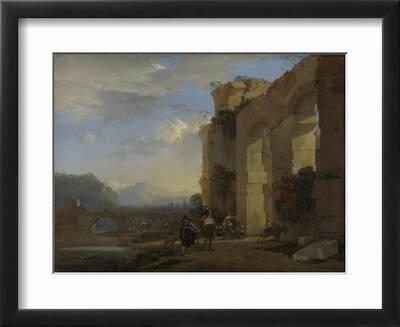This is a framed painting, displayed within a black frame and white mat, showcasing a picturesque and somewhat blurred scene. The painting seems to be a watercolor and depicts an ancient, possibly ruined structure, which could be an aqueduct bridge or a castle with arched openings. The setting features a cloudy, predominantly blue-gray sky, with the Sun possibly rising over distant mountains. In the foreground, there are a couple of indistinct figures, one of whom might be on horseback, along with a large, bushy tree. The scene also includes a bridge crossing a stream or river. The color palette consists of muted tones and tans, except for the blue of the sky, lending it a subdued, vintage appearance.